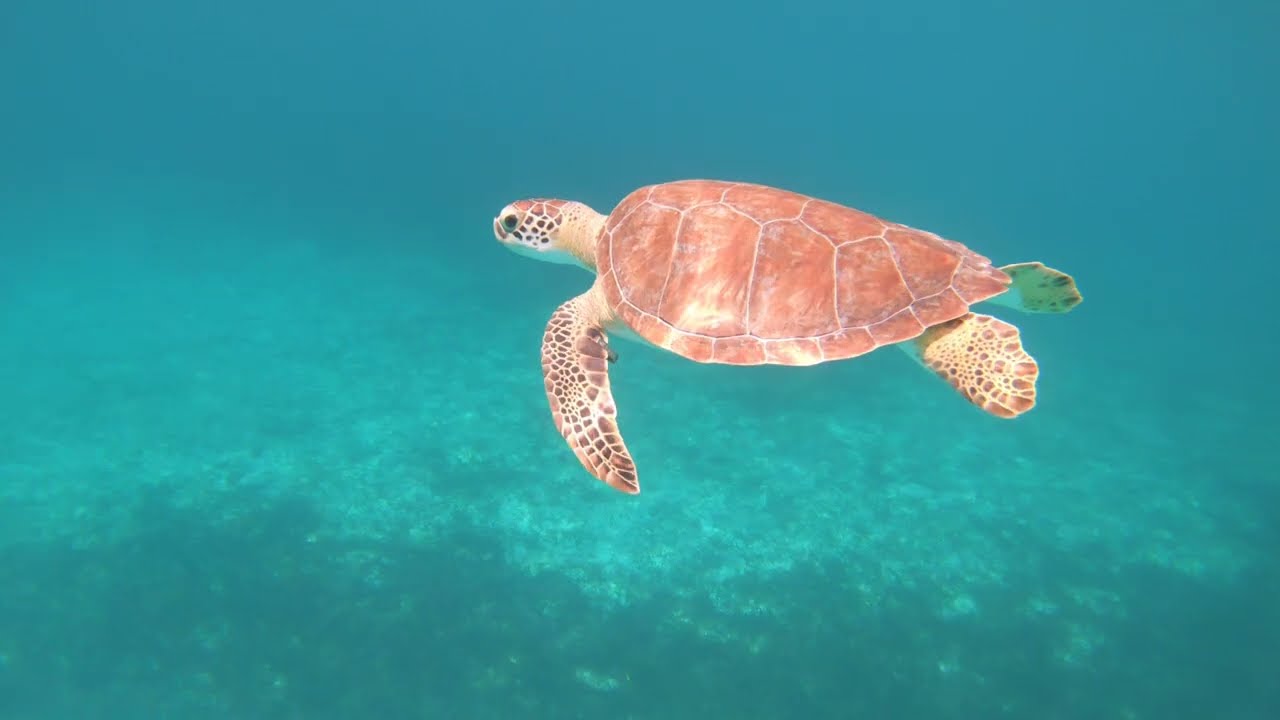This detailed photograph captures a majestic giant sea turtle swimming gracefully from right to left in a vibrant, teal-blue ocean. The turtle's peach and yellow shell is intricately marked with lines and patterns, and its scaly front feet propel it forward. Its head features brown dots on a green background, and a clear black eye is prominently visible. The turtle's brownish back and front fins, adorned with tiny black and brown spots, add to its distinctive appearance. Surrounding the turtle, the sea water varies in color, transitioning from a deep, darker shade at the bottom to a lighter, more aqua hue near the surface. The rocky formations on the ocean floor are faintly visible, enhancing the natural underwater setting. The image beautifully showcases the turtle's side profile as its head juts forward, embodying both the age-old wisdom and serene beauty of these long-living creatures.